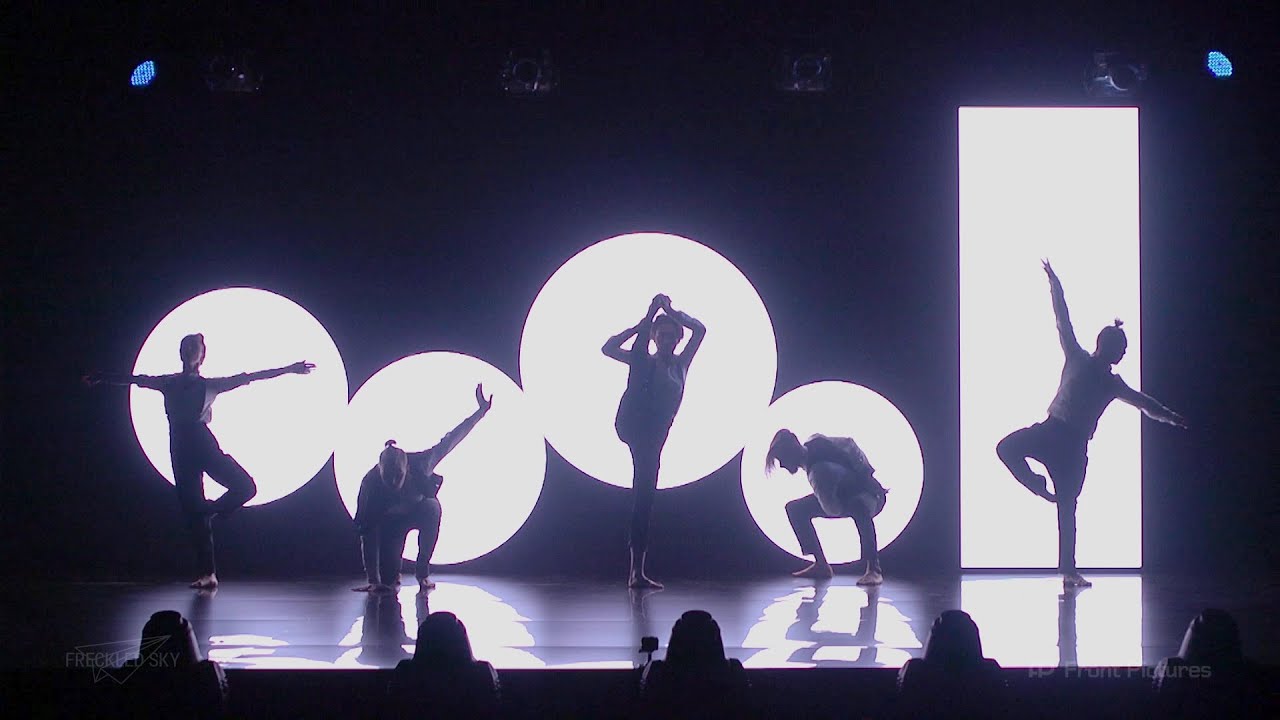This image captures a dynamic theater or dance performance set against a striking backdrop of bright, geometric lights. The stage is dimly lit overall, with the primary illumination provided by four intensely bright, circular lights arranged in an alternating high-low pattern, casting dramatic silhouettes of the performers. Additionally, the far-right performer is lit by a tall, rectangular light, creating a unique contrast among the figures. There are five dancers, each adopting a distinctive pose: the first dancer strikes a T pose with her left leg folded to form a figure-four shape; the second is in a superhero landing pose; the third showcases flexibility by holding her leg next to her ear; the fourth is crouched down, reaching an arm between her legs; and the fifth, illuminated by the rectangular light, assumes an elegant ballet pose with her right leg in a figure-four formation, one arm raised and the other extended to the side. The stage lights highlight the performers' silhouettes, with the configuration of lights framing each dancer beautifully and even the faint outlines of the front-row chairs visible, hinting at the audience’s presence.